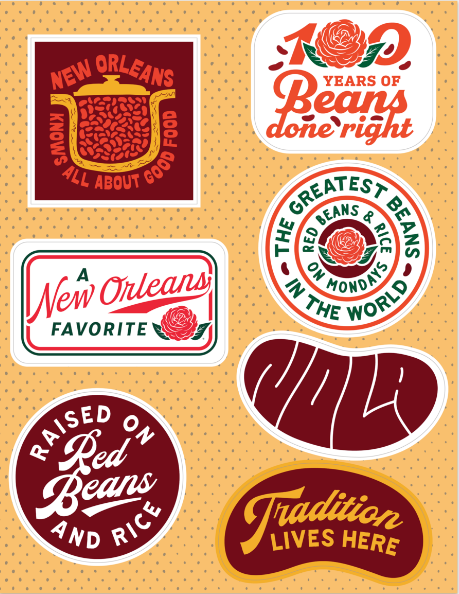This poster, with a vertical or portrait orientation, features a collection of emblems, logos, and badges arranged symmetrically against a dark orange, almost beige background. The backdrop is covered with uniformly spaced grey dots, creating a pegboard-like pattern. The various shapes of the emblems include a square on the top right, a sideways rectangle on the middle left, and a circle on the bottom left, accompanied by a curved-edged rectangle on the top right, another circle below it, and two kidney bean shapes, one on its back and one on its stomach, towards the right. 

Prominent emblems include:
- A top-left logo that reads "New Orleans knows all about good food," accompanied by an image resembling beans in a container.
- A hot dog-shaped badge on the bottom right with golden text proclaiming "Tradition lives here."
- A circular red logo to the left of this that states "Raised on red beans and rice."
- Another bean-shaped logo above it that simply says "NOLA."

Other text scattered across the emblems highlights phrases related to New Orleans' culinary heritage, such as "100 years of beans done right," "The greatest beans," and "Red beans and rice on Mondays." The emblem colors range from burgundy, red, and orange to various shades of white, complementing the poster's thematic hues. Among the visual elements are illustrations of orange-rimmed pots and kidney beans, underscoring the region's famous cuisine.